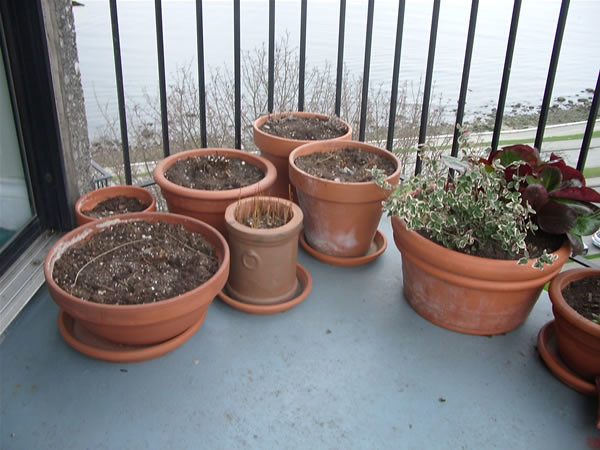The image portrays an elevated patio or balcony, likely part of an upper-story apartment. The flooring is a bluish-gray concrete with some dirt and markings. Spread across the patio are approximately seven to eight traditional clay flowerpots in terracotta color, many of which have saucers beneath them to catch water. Most of these pots are filled with soil and occasionally pebbles and fertilizer pellets, with some showing the very beginnings of plant growth. However, one larger pot on the right stands out with two distinct plants: one having small green leaves edged in white, and the other showcasing a mix of maroon, brownish, and greenish leaves. The patio is enclosed by thin black metal bars, and beyond this, a serene body of water is visible, likely a lake or river, bordered by bare trees and a roadway. Additionally, there's a sliding door or window frame visible to the left, confirming the setting as an outdoor space attached to a living area.